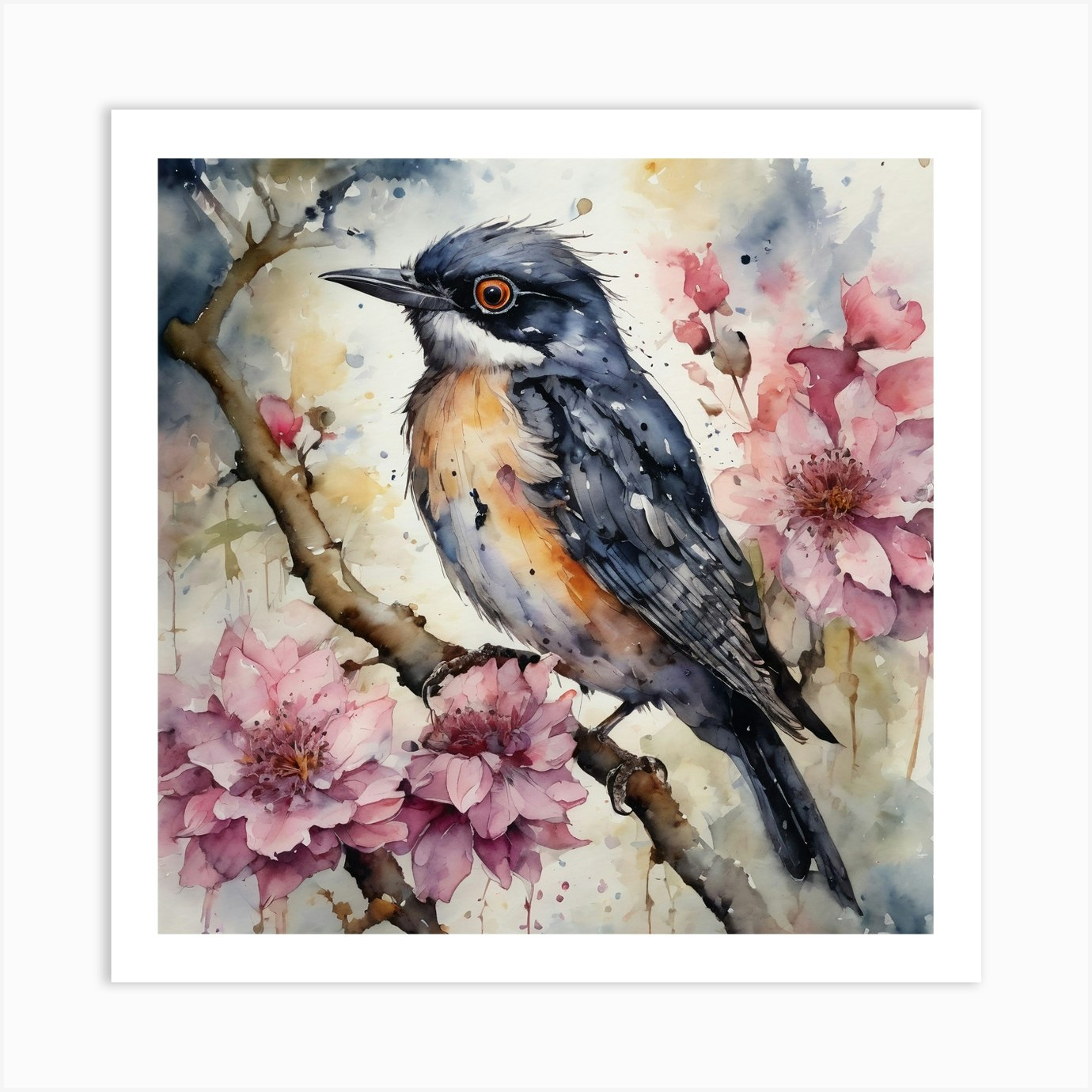This watercolor painting features a detailed and realistic depiction of a Baltimore Oriole perched on a tree branch, set against a pastel-muted background. The oriole, central to the composition, faces left and displays a striking combination of black feathers on its head and wings, a rusty brown chest, and a white belly. It has an orangish-red eye and a long, narrow dark gray beak. The bird's feet grasp a slender branch that extends diagonally from the lower right to the upper left of the image. Surrounding the bird are delicate pink flowers with darker pink and white accents, including two prominent flowers on the left and one on the right behind the bird, along with several smaller unopened buds. The background is a soft blend of yellow, gray, and blue watercolor washes, harmonizing with the overall muted tones. The painting is presented within a white matting, emphasizing its rectangular shape, and exudes a tranquil and charming aesthetic.